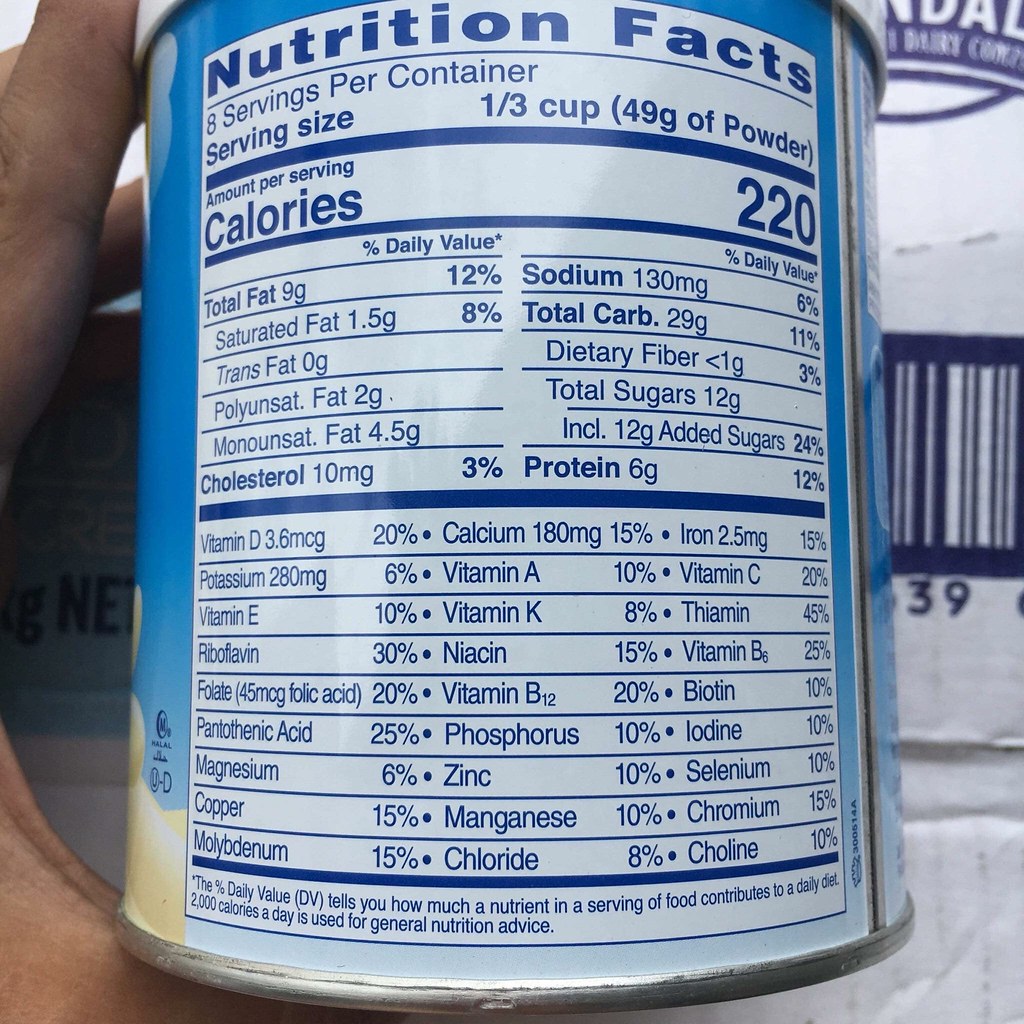An up-close image captures a nutrition label on a cylindrical canister. A white male hand is holding the canister on the left side of the frame; the curvature of the hand, including the pointer finger at the top and the thumb underneath, is clearly visible. The label prominently displays nutritional information: 8 servings per container, with each serving size being 1/3 cup or 49 grams of powder. Key nutritional facts include 220 calories and various fat contents: total fat at 9 grams (12% DV), saturated fat at 1.5 grams (8% DV), along with trans fat and polyunsaturated fat information. The label also lists protein and calcium, noting calcium content specifically at 180 milligrams (15% DV), among other nutrients.